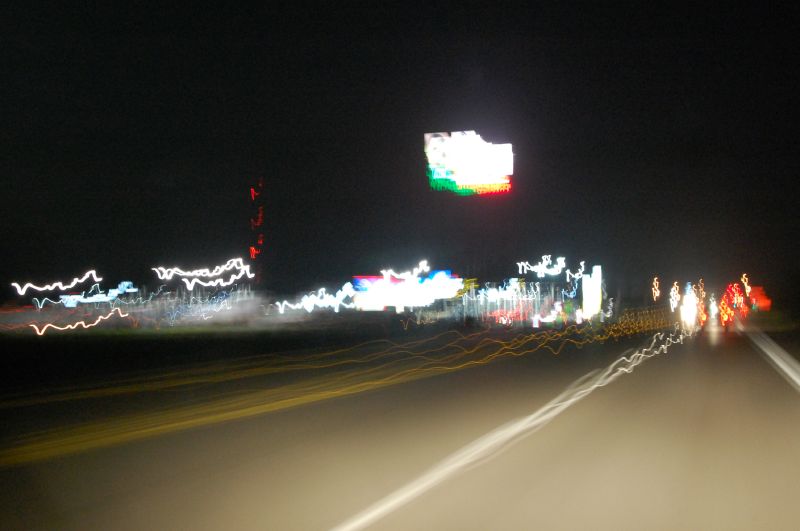A nighttime photo taken from a car dashboard on a dark road illuminated by various lights. The scene is wrapped in complete darkness, punctuated by a variety of blurred and elongated lights that streak across the image. The yellow and white lines on the road appear disjointed and smeared, creating an almost ethereal effect. To the right, a series of similarly streaked and indistinct lights suggest the presence of a shopping center or city, with a prominent, but indecipherable, billboard that might belong to a hotel. On the left side, additional blurred lights hint at the headlights of another vehicle in the distance. The overall image is a chaotic mix of red, white, green, and more, making it nearly impossible to discern any specific details, but effectively conveying the sense of motion and the vibrant, disorienting nature of nighttime driving.